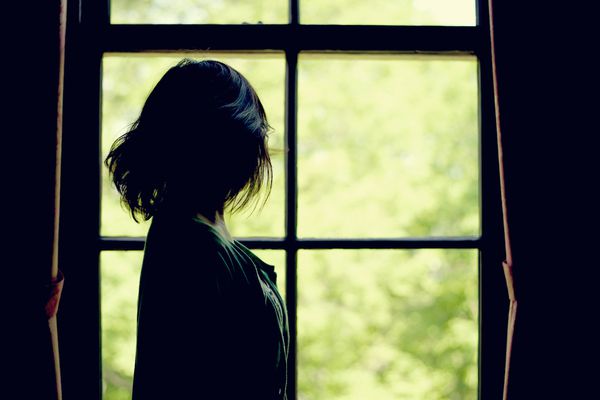This photograph captures a teenage girl in profile, standing against a brightly lit window that casts her mostly into silhouette with subtle highlights edging her form. She has shoulder-length, layered brown hair and is clad in drab-colored clothing, potentially a dress paired with a sweater. The girl is positioned on the left side of the window, gazing outward. The window itself comprises four bottom panes on the movable part and partial views of two upper panes. Framing this scene are two reddish curtains, each tied back to reveal the window and the blurred greenery outside, likely from a large sunlit tree. This backlit composition emphasizes the contrast between the bright exterior and the darker, nearly monochrome foreground.